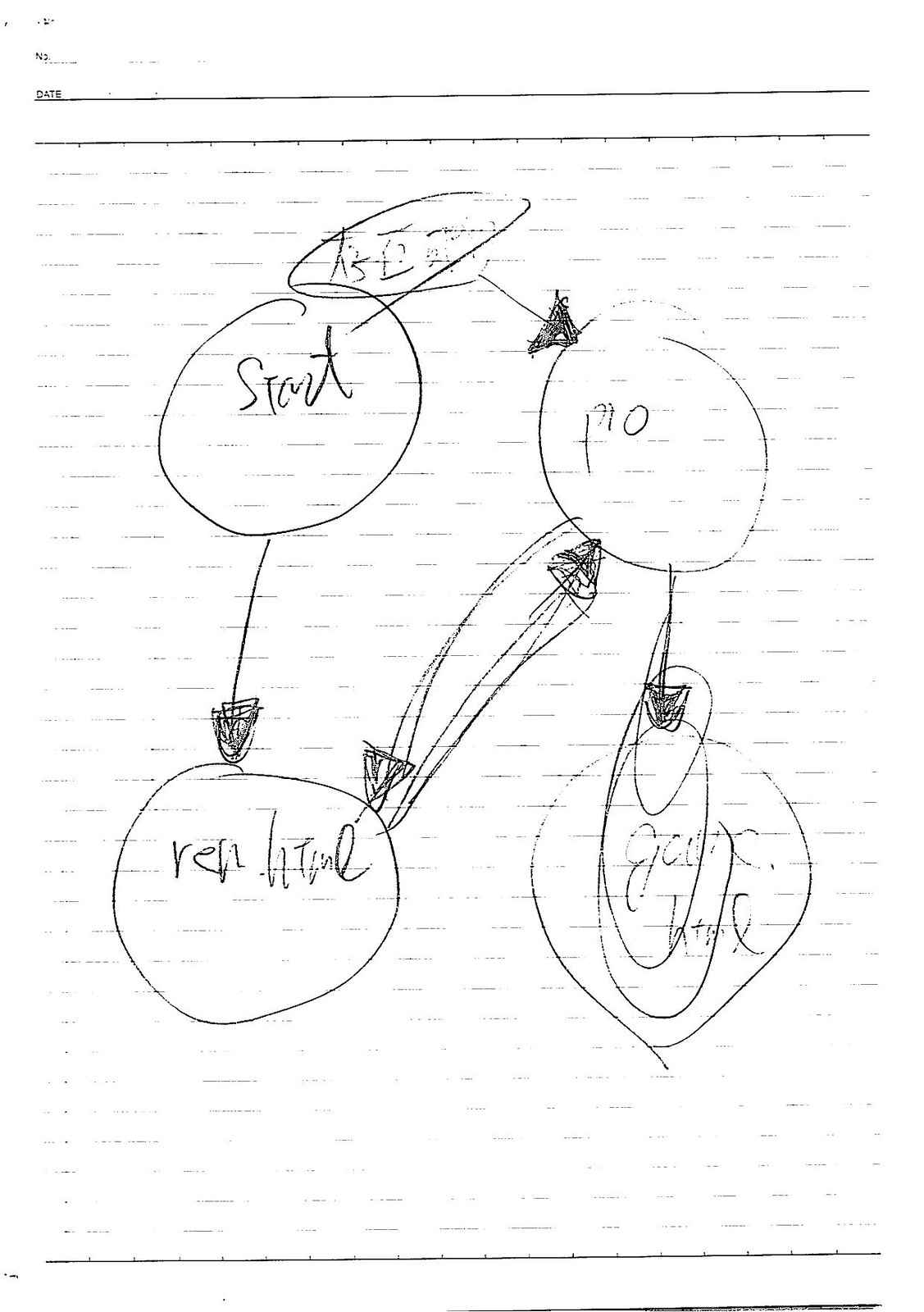A detailed black and white image showcases a hand-drawn diagram on a lined background, likely white paper. The background features horizontal lines, with two prominent lines across the top, one complete line at the bottom, and another partially visible lower line at the base. The image appears to be a photocopy or a hand-drawn representation, adding to its rustic charm.

At the core of the diagram are five circles, each connected by arrows, resembling a flowchart or infographic. The circles contain various inscriptions in scribbled handwriting. Starting from the top left, the first circle appears to read "Strut" or "Stout." Directly above, a second circle contains the letters "G-E-R." A thick, filled-in arrow directs the flow from this circle to a third circle on the upper right, labeled "F-O."

Below these, a fourth circle sits in the lower left quadrant, seemingly inscribed with the letters "R-I-V." The fifth circle, positioned at the lower right, includes the characters "G-O-C" and possibly an "L," and is filled with several smaller, scribbled circles within its perimeter.

Arrows map the relationships between these circles. One arrow moves from the top left circle to the lower left circle, while another links the upper right and lower left circles bidirectionally. Finally, an arrow connects the top right circle to the lower right circle. The overall design suggests connectivity and flow between different yet interconnected components.